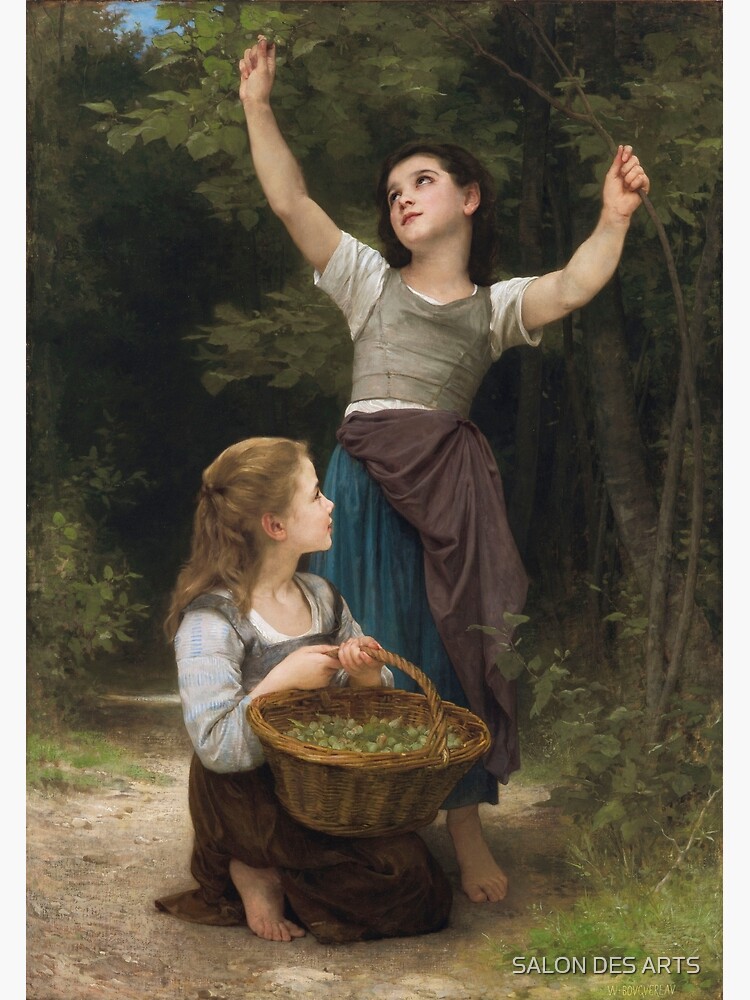The image depicts two young girls in a dense forest setting, seemingly around 11 or 12 years old, both dressed in simple attire. The girl on the right is standing barefoot on a dirt pathway, wearing a white and gray t-shirt under a long blue dress, with a shawl around her waist. She is pulling down a branch with her left hand while reaching to pick flowers or small green fruits with her right hand. Meanwhile, the girl on the left is kneeling on the same earthen path, also barefoot, in a similar white and gray shirt paired with a long brown dress. She holds a woven brown basket containing green leaves or possibly small green fruits, like unripe berries. Both girls are focused on their task, with the kneeling girl looking up at the standing one, who is busy gathering the natural items from the branch. The scene is set against a backdrop of thick foliage and trees, characteristic of a dense forest, with a dirt pathway meandering through. A watermark in the lower right corner reads "Salon des Arts," indicating the artistic nature of the depiction.